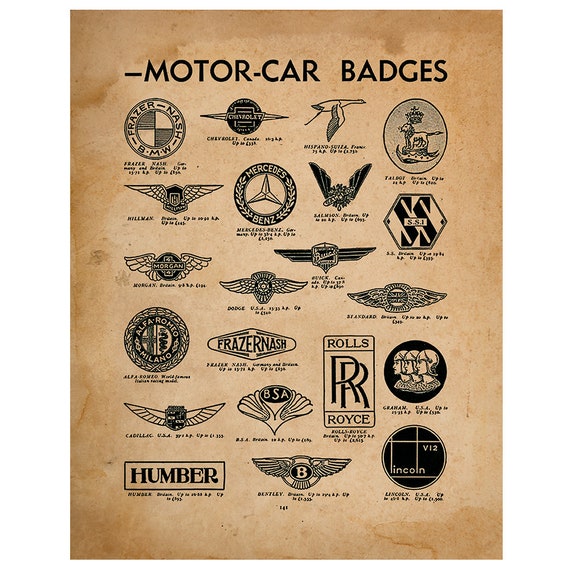The image depicts an aged graphic or poster, originally white but now browned and water-stained, especially along the edges. The background is busy with black text and numerous small and intricate insignias. The poster is titled "Motor Car Badges" prominently at the top. Displayed across the sheet are over a dozen badges for various automobile companies, each labeled beneath with finer print that's difficult to read. Among the recognizable emblems are those of Rolls-Royce, BMW, Mercedes, Lincoln, and Humber. The badges vary in design—some are winged, some circular, some crests, and others resemble birds, invoking the look of pilot wings. Despite the lack of color, the detailed black illustrations on the off-white, weathered paper showcase these historical auto insignias in an intricately arranged and meticulously labeled fashion.